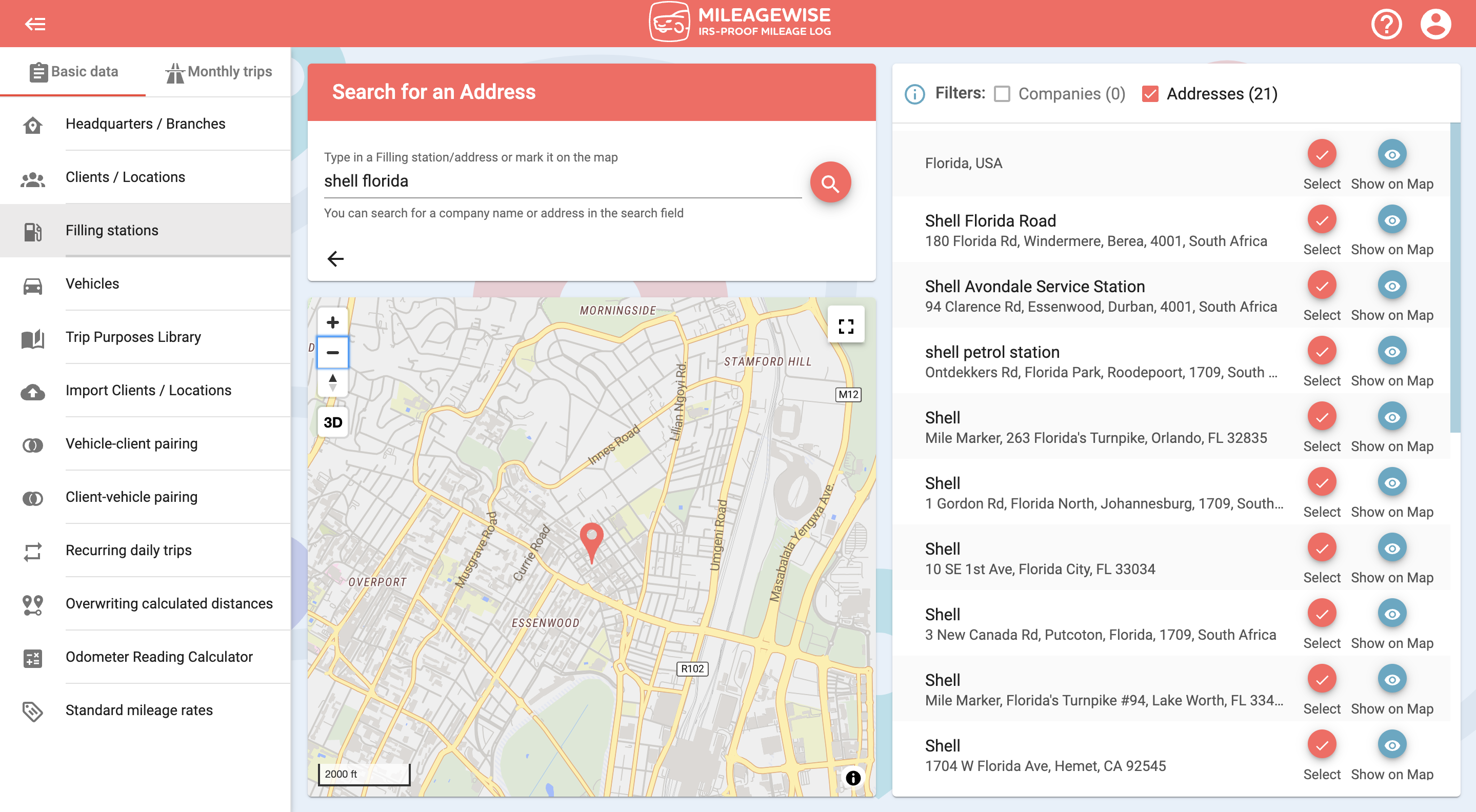The image is a screenshot of a page from the MileageWise application. The header at the top of the page is a distinctive shade, blending between pinkish red and pink, and features the company’s branding. At the center of the header, the name "MileageWise" is displayed in bold white capital letters as one word. To the left of the company name, the logo is present: a simple white outline of a square with rounded corners and a minimalist sketch of a car's front view.

Beneath the header, the tagline "IRS Proof Mileage Log" is also presented in white font. In the upper right corner of the page, there are icons for account access and help—a generic account symbol and a white question mark inside a white circle, respectively.

In the main section of the application, there is a white rectangle banner that reads "Search for an address" in white font. The address currently selected is "Shell, Florida," and below this, a map is displayed with a location marker indicating the selected address.

On the right side of the screen, the search results related to the query are visible, listing various addresses for Shell gas stations, such as "Shell Florida Road" and "Shell Avondale Service Station," with additional entries continuing beyond the visible area.

To the left side, a sidebar contains a vertical list of menu items in gray font. These options include "Headquarters/Branches," "Clients/Locations," "Filling Stations," "Vehicles," "Trip Purpose Library," among others, which represent the various utilities available for users within the MileageWise platform to efficiently track their mileage.